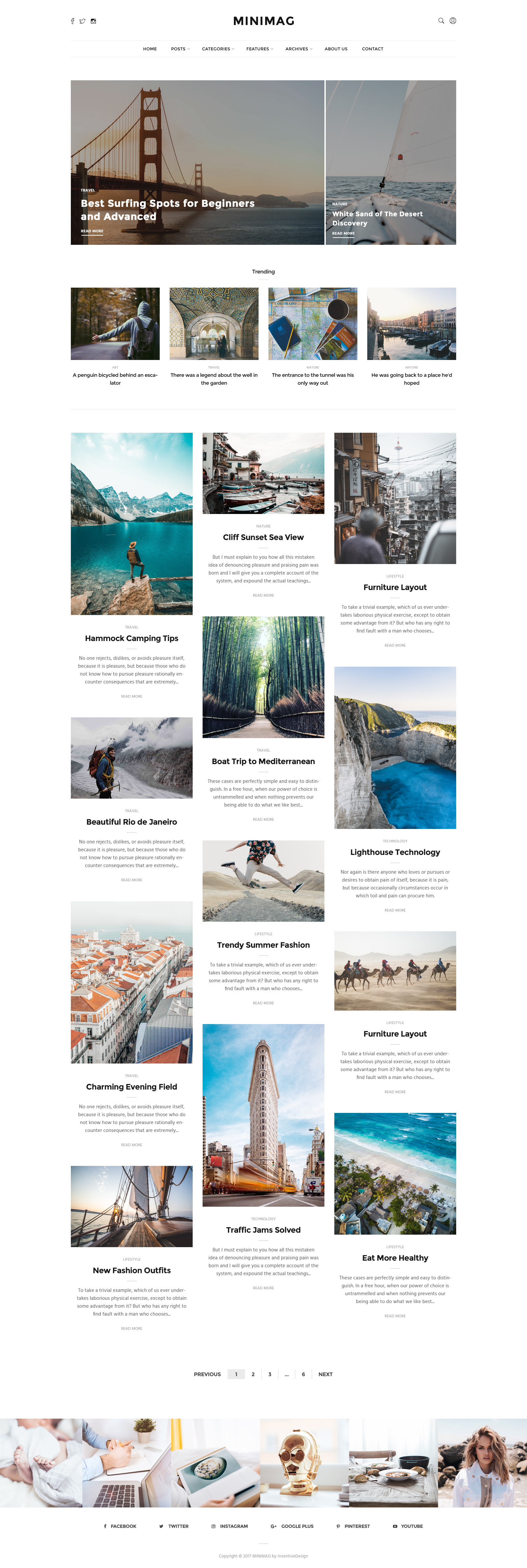Vertical website layout on a smart device showcasing a modern, interactive interface:

- **Header**:
  - **Top-Left Corner**: Icons for Facebook, Twitter, and Instagram.
  - **Center**: The bold, black, uppercase text "MINIMAG".
  - **Top-Right Corner**: A magnifying glass icon (search function) and a generic user profile icon.

- **Navigation Menu**: 
  - Positioned just below "MINIMAG".
  - Encapsulated by gray lines and features clickable black, uppercase categories: HOME, POSTS, CATEGORIES, FEATURES, ARCHIVES, ABOUT US, and CONTACT.

- **Main Content**:
  - Below the navigation menu, an array of articles with images.
    - **First Article**: Image of the Golden Gate Bridge titled "Best Surfing Spots for Beginners and Advanced".
    - **Second Article**: Image of a nature scene titled "White Sand of the Desert Discovery" with a "Read More" link.
    - **Trending Section**: Highlighted articles including:
      - A penguin riding a bicycle behind an excavator.
      - A legend about a well and a tunnel wall's entrance being someone's only way out.

- **Footer**:
  - Pagination showing "Previous", "1" (highlighted in gray), "2", "3", "...", "6", and "Next" for navigation.
  - Additional images and social media links for further engagement at the very bottom of the page.

This comprehensive layout provides a clear, engaging format for users to explore various categories, articles, and social media platforms.